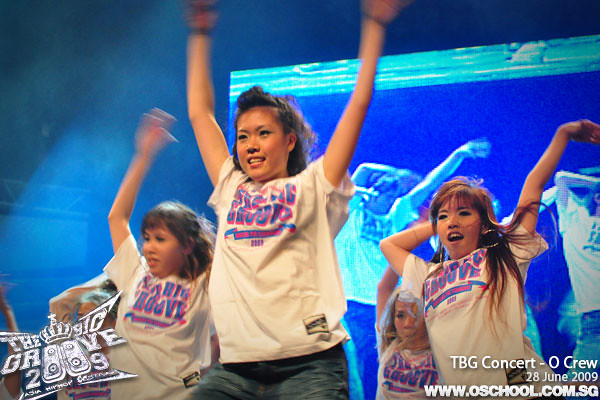The image captures a group of four Asian teenage girls dancing indoors, centered in front of a large blue screen displaying a video of other dancers. Each girl is dressed in a white t-shirt adorned with large blue lettering outlined in pink and a blue banner with pink text. They appear to be moving in unison with their hands raised. The scene is likely part of a music concert or dance event as indicated by the text overlay in the bottom corners. The bottom left displays a white logo possibly depicting a crown and speakers with the partially readable text "Magic Groove 2009." The bottom right includes the event details: "TBG Concert, Okru, 28 June 2009, www.oschool.com.sg." The setting, with its palette of light blue, dark blue, white, pink, purple, and gray, suggests an organized and lively performance atmosphere, typical of Singaporean cultural showcases.